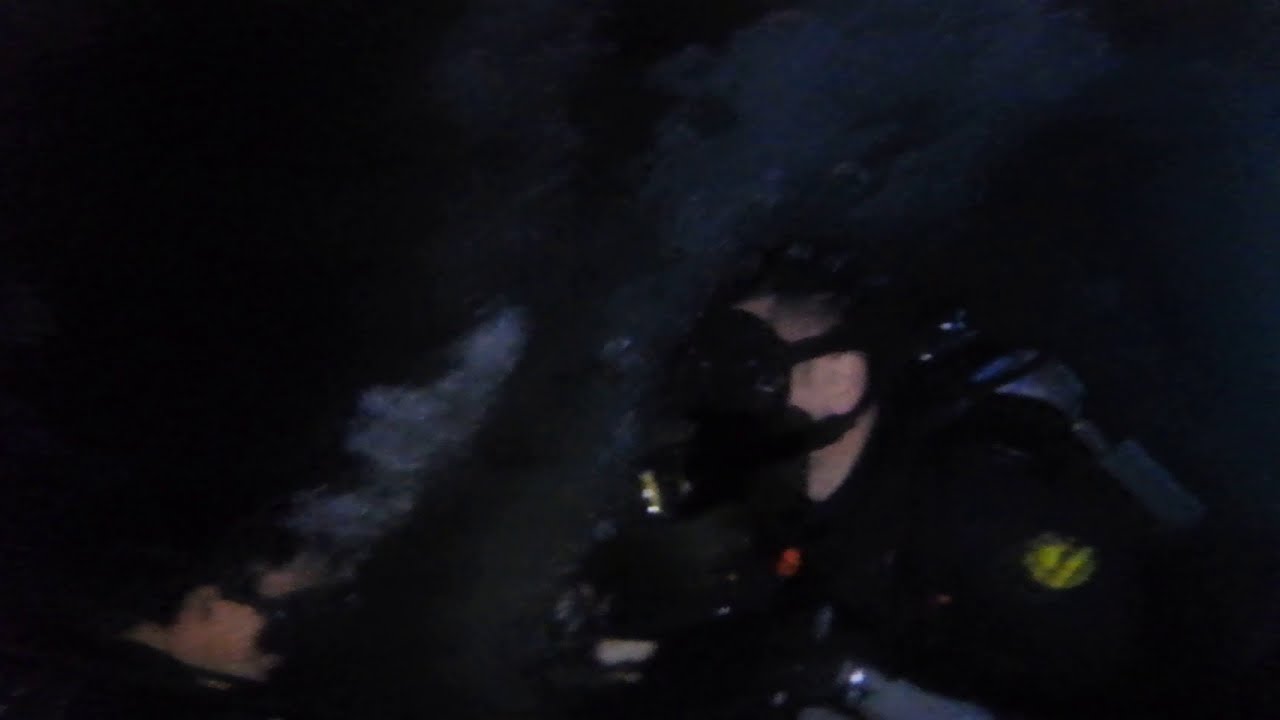The image depicts a dimly lit underwater scene featuring a single figure viewed from the head down to almost the waist. The individual is wearing a scuba mask that covers the eyes completely and has an oxygen tank strapped to their back. The person appears to have short white hair and is dressed in a dark jacket or shirt with potential patches or insignias, though details are obscured due to the darkness and blurriness of the shot. There's a noticeable patch of green on the shoulder, and a red area around the neck, possibly indicating additional gear. Bubbles emanate from the breathing apparatus, adding to the murky atmosphere. On the left side of the scene, partially outlined, is what looks like a hand holding the scuba mask, enhancing the impression of a deep underwater environment filled with darker hues of blue and sporadic clouding. Despite the low light and shadows, the elements combined suggest the person is exploring an underwater space, possibly on a challenging night dive.